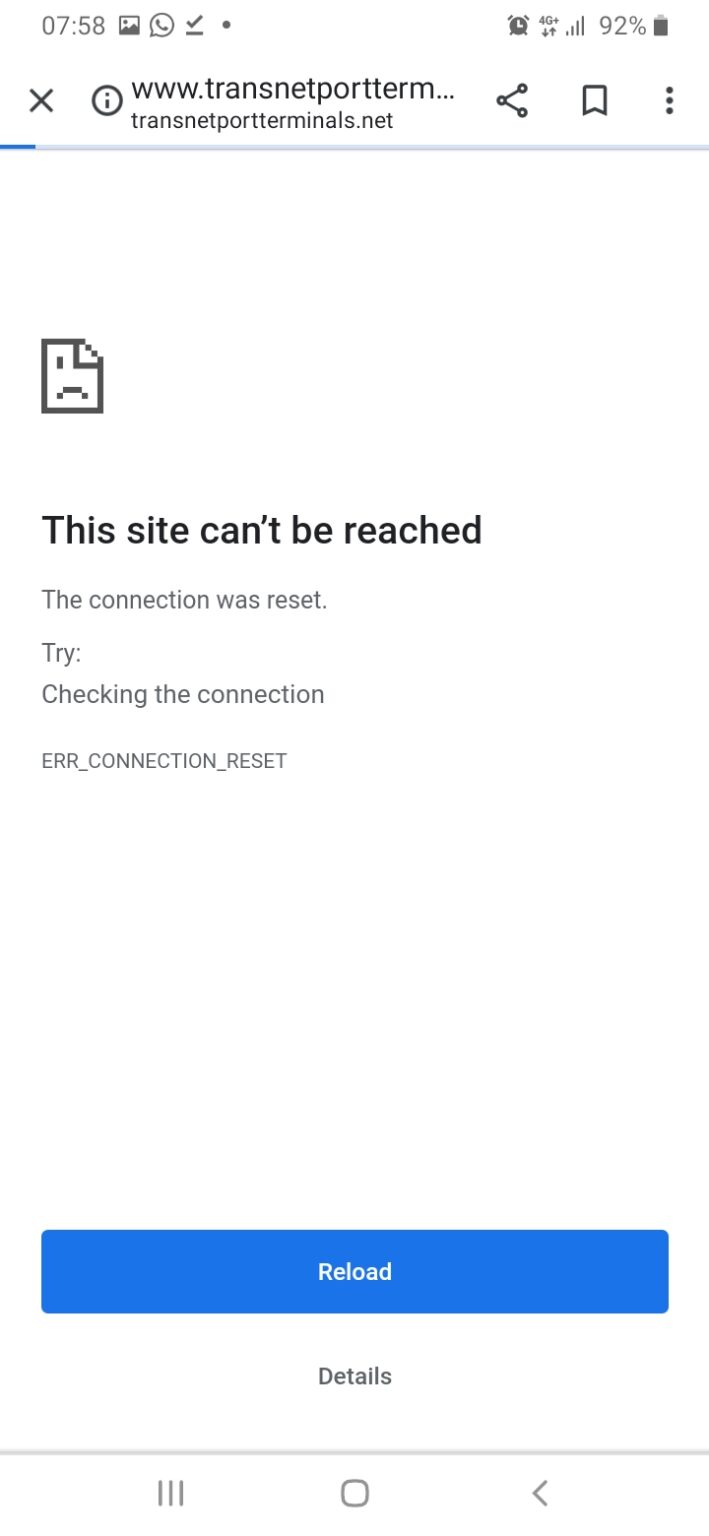The image showcases an iPhone displaying a webpage with the URL "www.transnetportterm.net." The phone's status bar indicates a 92% battery charge, and the time shows 7:58. The browser interface includes various icons at the top: a circle with an 'i' symbol, a generic 'X' icon, an internet connection indicator, a box, and three vertical dots.

Below these icons is a progress bar with a faint blue tint on the left side, suggesting it is a loading bar that has barely advanced. Dominating the screen is an unfortunate error message featuring an image of a folded box with a sad face on it. Large black text reads, "This site can’t be reached,” followed by smaller text stating, "The connection was reset. Try checking the connection. ERR_CONNECTION_RESET."

At the bottom of this message, there is a blue button labeled "RELOAD," and underneath that a smaller "Details" link. The screen is capped with a light gray line separating it from the browser's bottom interface, which includes three vertical lines, a square likely representing the home button, and a left-pointing arrow for navigating back.